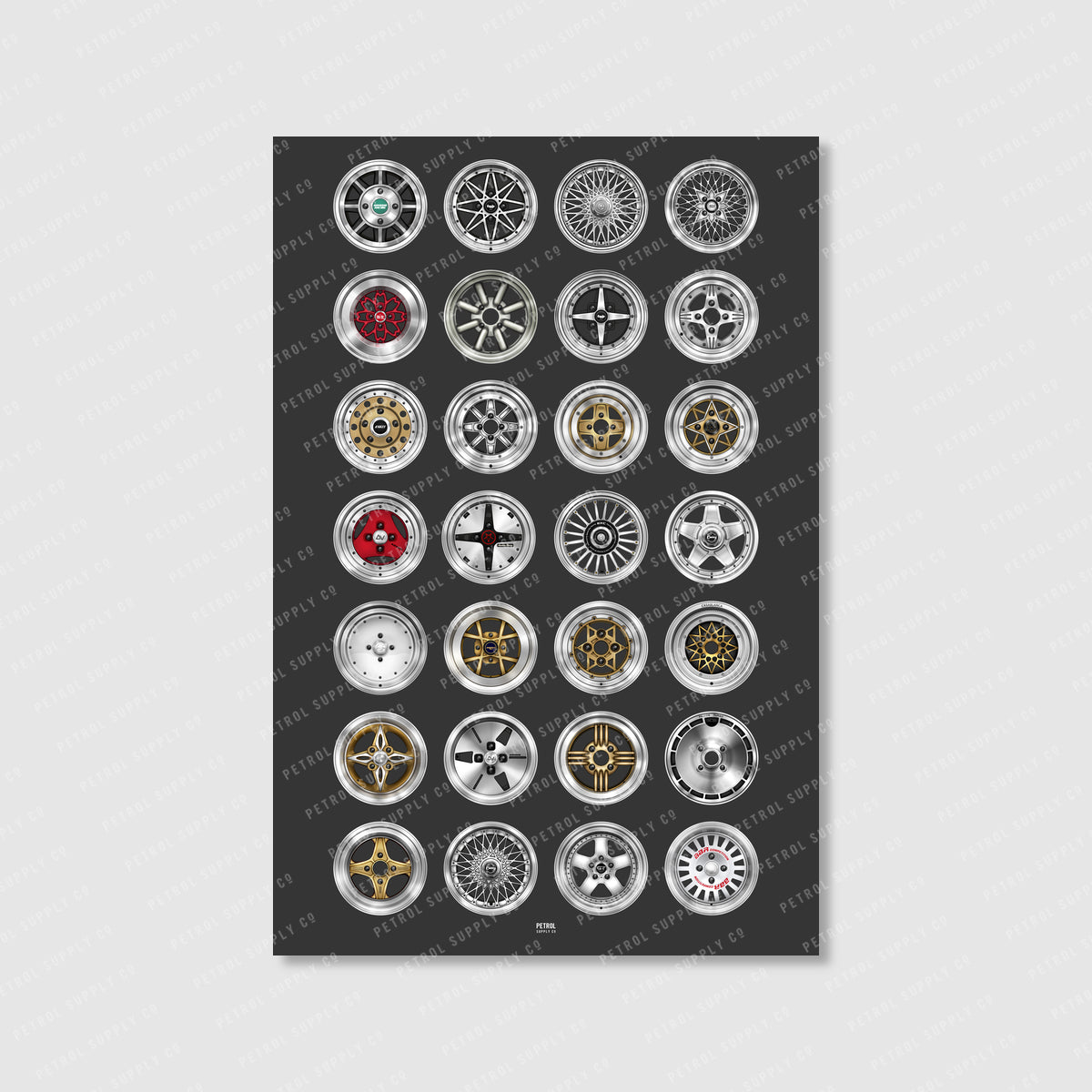The image features a dark gray background with a prominent darker gray, almost black, upright rectangle situated within it. This central rectangle displays a grid comprising 28 artistically decorated hubcaps, laid out in 4 columns and 7 rows. Each hubcap exhibits a distinct design, embodying an array of silver, gold, black, and red accents. The designs vary immensely, featuring minimalistic patterns with just a few spokes, to intricate, nearly solid interiors with small center dots. One notable hubcap at the top boasts a green dot at its center, while another towards the top-right corner showcases teardrop-shaped spokes. Behind this grid of hubcaps, a diagonal repeating text reads "Petrol Supply Co." in a shadowy grey font, enhancing the industrial theme of the artwork.